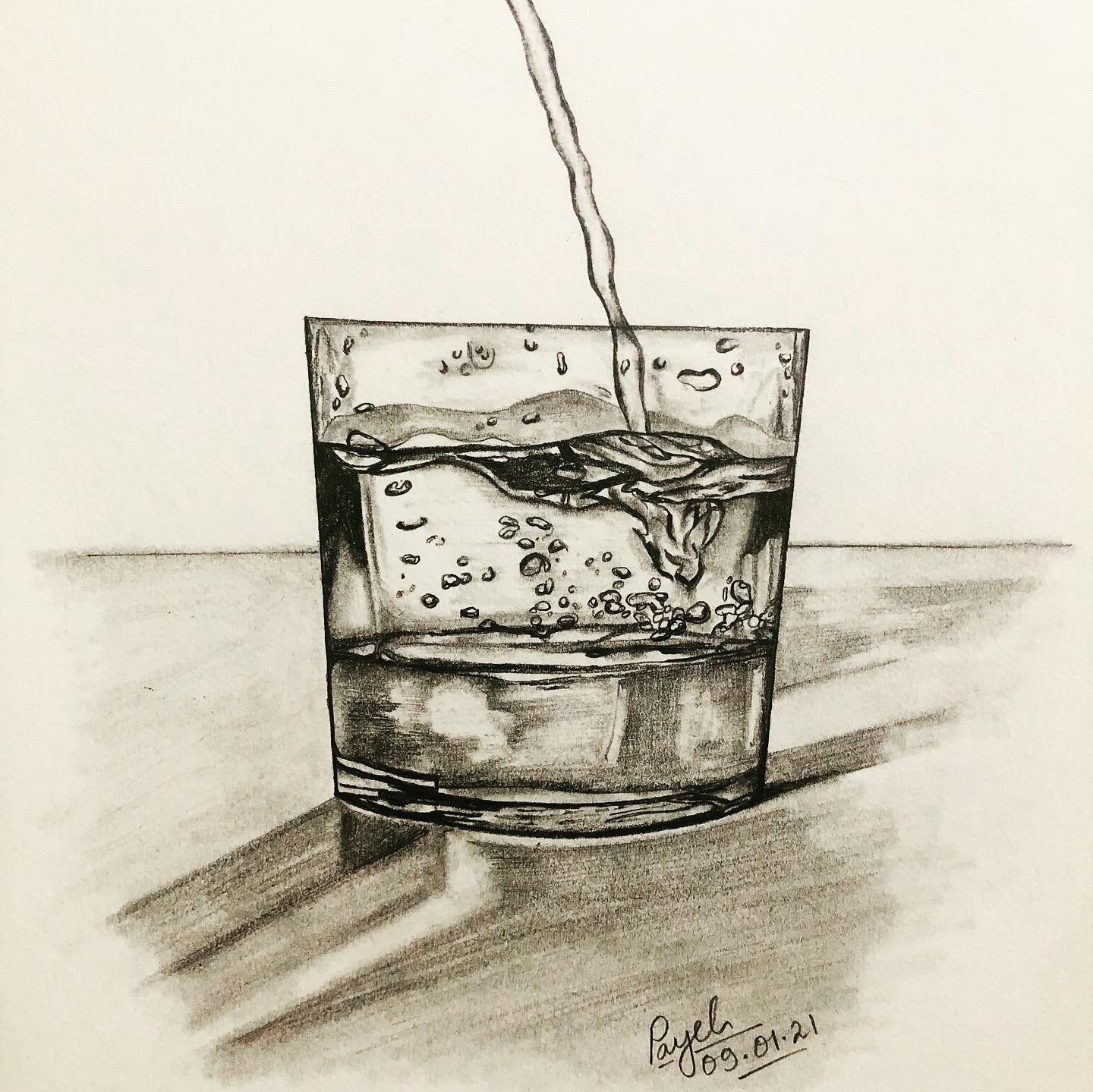This drawing, rendered in black pencil on an off-white square canvas, beautifully captures the simple elegance of everyday life. At its center is a meticulously detailed cup, placed on a table, into which a stream of liquid gracefully pours from the top left corner of the composition. The artist has skillfully employed shading techniques to create realistic shadows, emphasizing the cup's three-dimensional form and its position on the table. In the bottom right corner, the artist's signature is prominently displayed, accompanied by the date, "9-1-21," preserving the creation's temporal context.